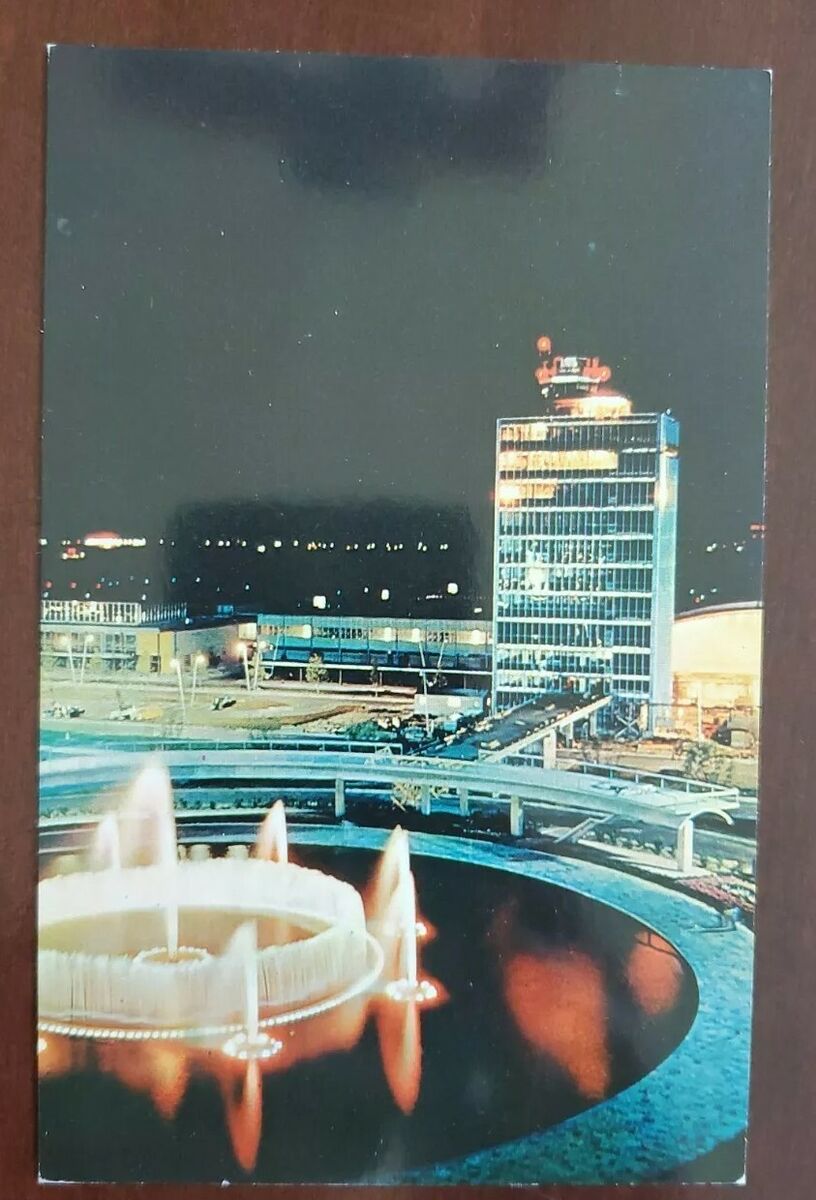The image shows a vintage-styled, color photograph displayed on a dark brown wall. The photo captures an urban nighttime scene featuring a large circular fountain with a calm pool at its base. Multiple spouts project water upwards, with the fountain illuminated by the orange lights reflected in the water. In front of the fountain stands a metal canopy with a platform on top, leading to a bridge that extends outward. This bridge connects to a towering skyscraper on the right side of the picture, with a radio tower atop it. The top three floors of the skyscraper are brightly lit, and city lights are visible in the distance to the left, contrasting against the grayish-green nighttime sky.